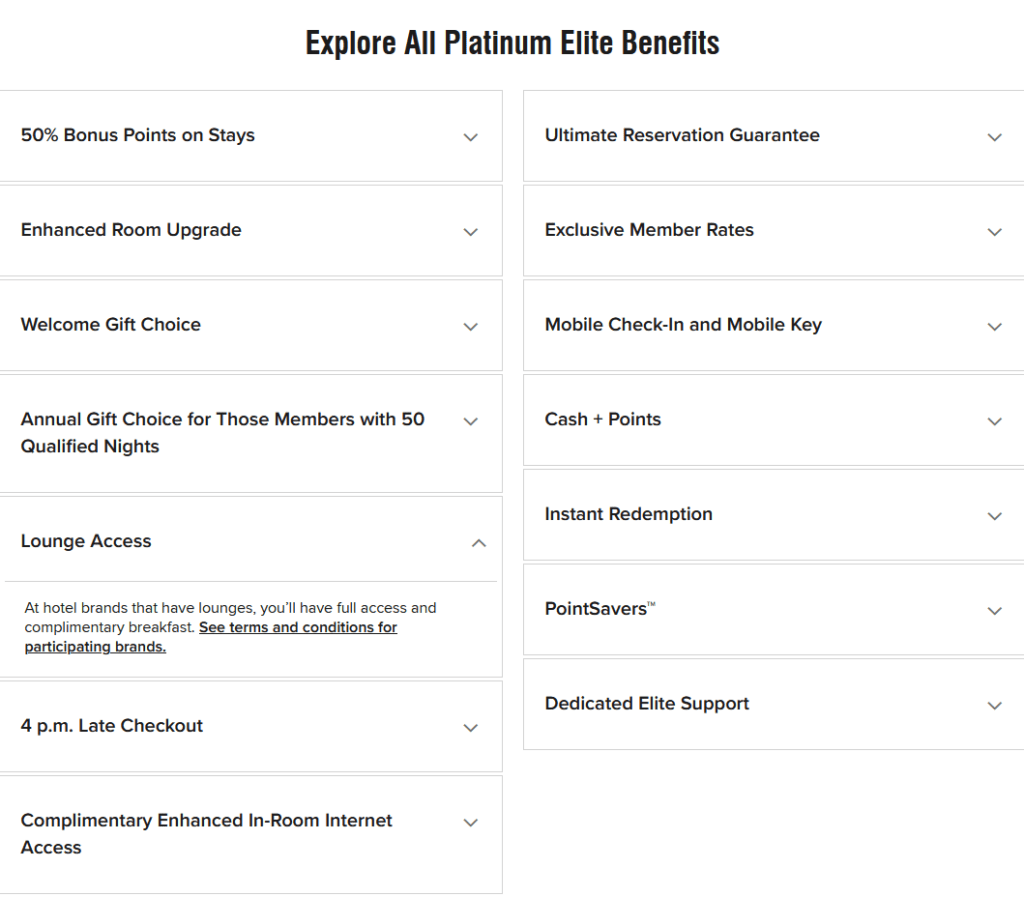The image depicts a webpage with an all-white background, featuring tabs on both the left and right sides. Across the top, a bolded black headline reads "Explore All Platinum Elite Benefits." 

On the left side, there are eight rectangular tabs with a light gray border and small separations between each. The tabs list the following benefits:
1. 50% Bonus Points on Stays (with a dropdown arrow on the right side of the tab).
2. Enhanced Room Upgrade.
3. Welcome Gift Choice.
4. Annual Gift Choice for Members with 50 Qualified Nights.
5. Lounge Access (with small black lettering underneath that states, "At hotel grounds with lounges, you have full access" followed by "Complimentary breakfast. See terms and conditions for participating brands," with the last line highlighted).
6. 4 PM Late Checkout.
7. Complimentary Enhanced In-Room Internet.

On the right side, there are seven rectangular tabs:
1. Ultimate Reservation Guarantee (with a dropdown arrow on the right side of the tab).
2. Exclusive Member Rates.
3. Mobile Check-In and Mobile Key.
4. Cash + Points.
5. Instant Redemption.
6. Points Savers.
7. Dedicated Elite Support.

At the bottom of the image, there is a small open space.